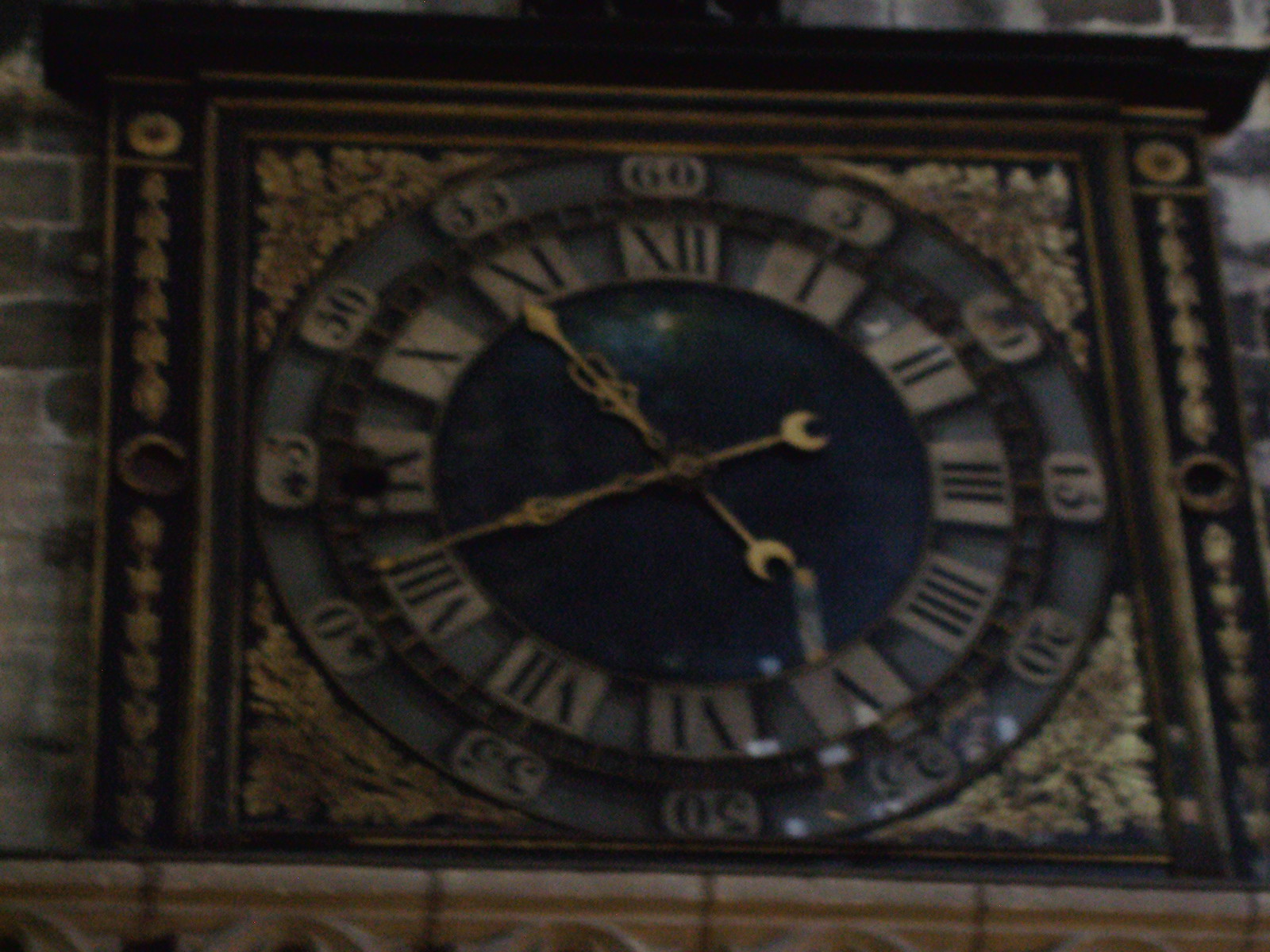The photograph captures a large, ornate outdoor clock affixed to the side of a brick building. The clock is enclosed in a square frame with intricate wood and black detailing, featuring gold carvings on the left and right sides. Each side of the frame displays a circular motif at the top and middle, with a square-like design running down the vertical line. The clock itself has a two-layer design: an outer circle with Arabic numerals in increments of five for the minutes, and an inner circle showcasing Roman numerals for the hours. The inner circle is predominantly black, adorned with two large golden hands that indicate the time. The clock's elaborate design, featuring a combination of gold, black, and brown hues, suggests it is a prominent fixture, possibly on a church or municipal building. The surrounding structure includes grayish-tan-brown bricks and a brown stone ledge, further emphasizing the clock's architectural significance.